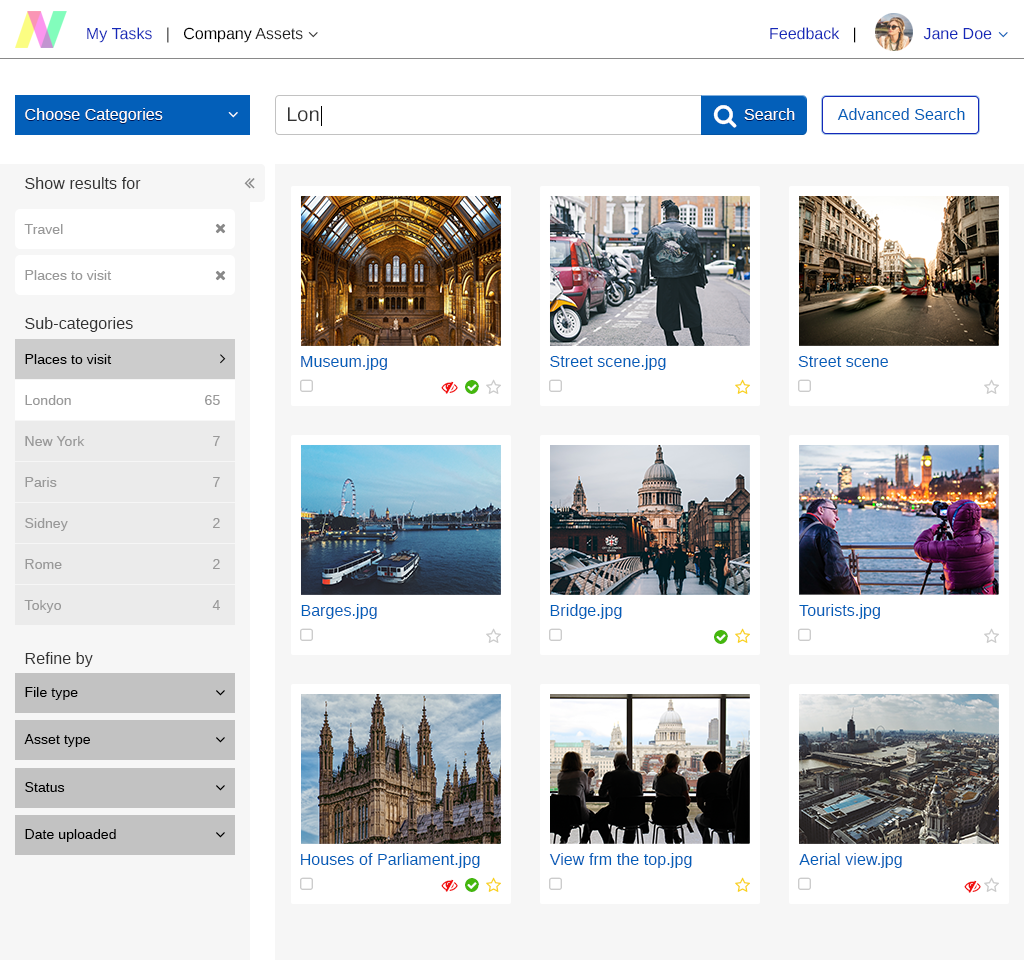**Detailed Caption:**

This is a large, square image depicting a well-organized digital user interface. At the very top, you see a colorful header displaying various overlapping shades of pink, yellow, and aqua. In the upper right corner, blue letters spell out "Tasks," and directly below this, black letters form the phrase "Company Assets" pointing downward with a "V" icon. Continuing in the upper right corner, blue letters read "Feedback," placed next to a vertical black bar. Adjacent to this is a circular avatar of a Caucasian female with long, round ponytail and sunglasses, identified as "Jane Doe" in blue letters next to a downward-facing "V" icon.

At the top center of the image, there is a search bar labeled with a blue search icon in white letters stating "Search" alongside a magnifying glass icon. Inside the text box, someone has typed "LoN," with a blinking cursor positioned after the "N." To the right of the search bar, there is a white box containing the blue text "Advanced Search."

Below the search bar are three rows of three thumbnail images, each depicting various scenes. 

- **First Row:**
  - On the left, an interior of an ornate museum, labeled "museum.JPG."
  - In the middle, a bustling street scene with cars, a motorbike, and a pedestrian, labeled "street scene.JPG," with a European city vibe.
  - On the right, an off-color street scene showing a double-decker bus, labeled simply "street scene."

- **Second Row:**
  - On the left, a riverfront scene with two low riverboats and a ferris wheel set against a clear evening sky, labeled "barges.JPG."
  - In the middle, a domed building resembling a capitol, labeled "bridge.JPG."
  - On the right, tourists in cold-weather attire, one taking a photo of the London skyline at night, captioned "tourists.JPG," showing landmarks such as Big Ben and the Houses of Parliament.

- **Third Row:**
  - On the left, the ornate upper structure of the Houses of Parliament under a partly cloudy sky, labeled "Houses of Parliament.JPG."
  - In the middle, silhouettes of four people gazing through a window, captioned "view from the top.JPG."
  - On the right, an aerial cityscape, labeled "aerial view.JPG."

Off to the left side of the picture, there is a text box that resembles a search bar, labeled "Choose Categories" in blue with white letters. Clicking on it reveals a long gray box with the options "Show results for travel" and "Places to visit." Subcategories listed are London (65), New York (7), Paris (7), Sydney (2), Rome (2), and Tokyo (4). Below these categories is a refinement section where users can toggle between file type, asset type, status, and date uploaded using clickable gray boxes with downward-facing arrows.